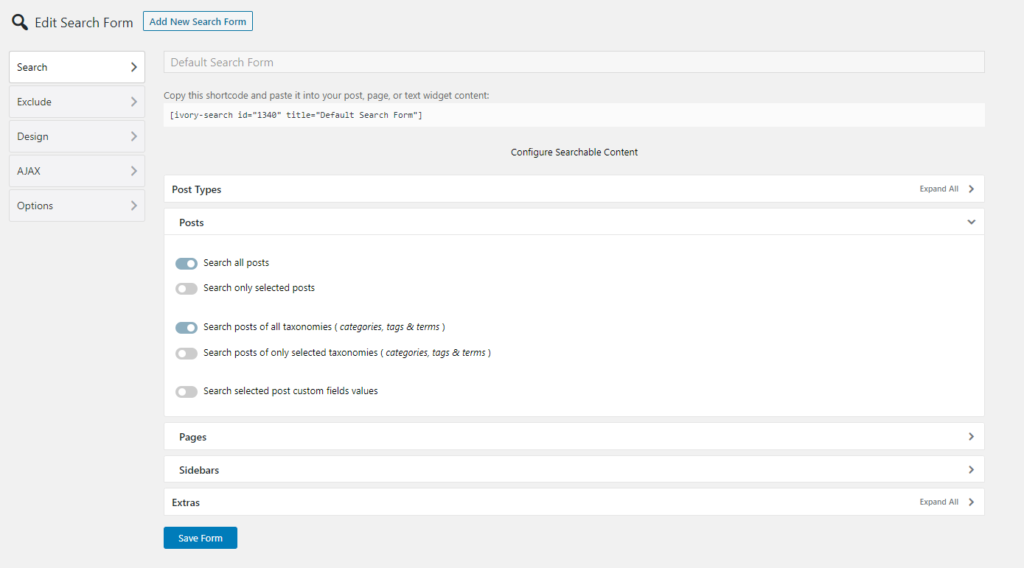The image displays a computer screen featuring a search form configuration interface. At the top, the options "Edit Search Form" and "Add New Search Form" are prominently displayed. The section labeled "Search Settings" is highlighted and includes options for a "Default Search Form." Users can exclude certain criteria and design their search forms as needed.

Further details reveal labels such as "AX" and "Siphons," along with a command to "Configure Searchable Context." In the main body of the form, a box titled "Post Types" allows users to refine their search. An arrow leads to a dropdown menu providing options to search all posts, selected posts, posts of all types, or posts of only selected types. Currently, "Search All Posts" and "Search Posts of All Types" are highlighted.

Beyond the "Post Types" section, additional categories include "Pages," "Sidebar," and "Extras," each with arrows indicating further options. The interface allows users to interact with these elements, make selections, and save their entries. A "Save" button is clearly visible, but the form does not present any identifying company information, leaving its origin unclear.